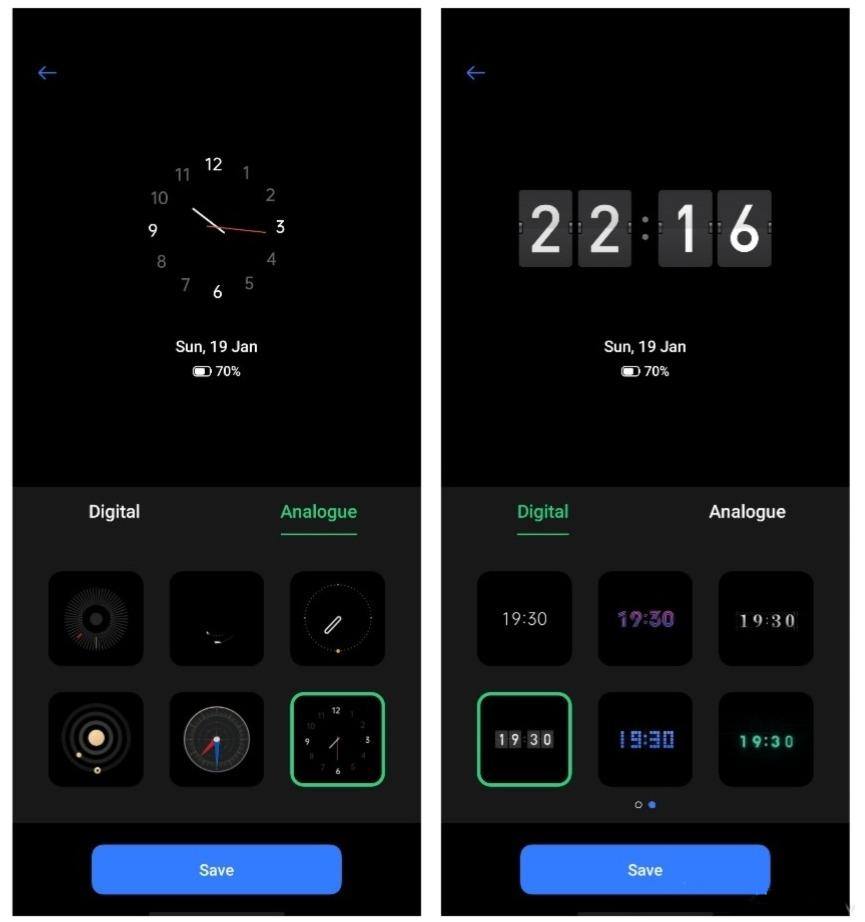The image is a screenshot showcasing an 'always-on display' customization interface. On the left side, there are options for analog clock designs, and on the right side, there are options for digital clock designs. Both sections feature six different clock designs each. The interface predominantly uses a black and green color scheme. At the bottom of the screen, there is a 'Save' button which allows users to apply their chosen clock design.